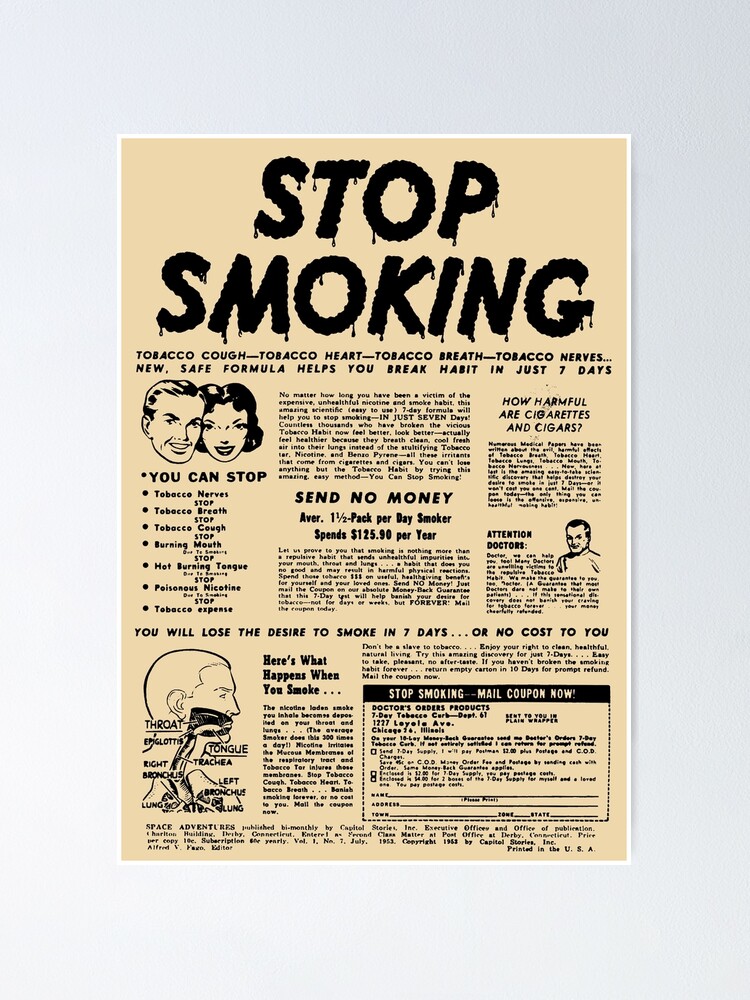This image is a reproduction of a vintage stop-smoking advertisement, likely from the late 1940s or 1950s, characterized by its old-school design and sepia-toned, dirty yellow background. At the top of the ad, bold black letters with a dripping effect spell out "STOP SMOKING." Below this, a series of slogans in smaller black capitals lists the detrimental effects of tobacco: "TOBACCO COUGH, TOBACCO HEART, TOBACCO BREATH, TOBACCO NERVES." The text promises a "NEW SAFE FORMULA" that helps break the habit in just seven days, emphasizing "NO COST TO YOU" if it doesn't work.

Beneath the slogans, there are stylized, black-and-white cartoon-like illustrations of a man and a woman. The provided tips and benefits for stopping smoking are listed around their images, including the cessation of "TOBACCO COUGH," "TOBACCO BREATH," "BURNING MOUTH," "HOT BURNING TONGUE," and "POISONOUS NICOTINE." There is also a section highlighting the financial savings of quitting, noting that the "AVERAGE 1.5 PACK PER DAY SMOKER SPENDS $125.90 PER YEAR."

On the left side, the ad features a detailed anatomical diagram, depicting the mouth, throat, esophagus, tongue, trachea, right and left bronchus, and lungs to illustrate the adverse effects smoking has on these body parts. This is accompanied by an explanation - though largely too small to read - of the physical health risks associated with smoking.

Towards the bottom section, it states "SEND NO MONEY" and includes a mail-in coupon labeled "STOP SMOKING MAIL COUPON NOW" from "DOCTOR'S ORDERS PRODUCTS," allowing users to fill out their name and address. This comprehensive anti-smoking poster provides various health warnings and offers a purported solution to quit smoking in an unusually detailed and visually compelling manner for its era.